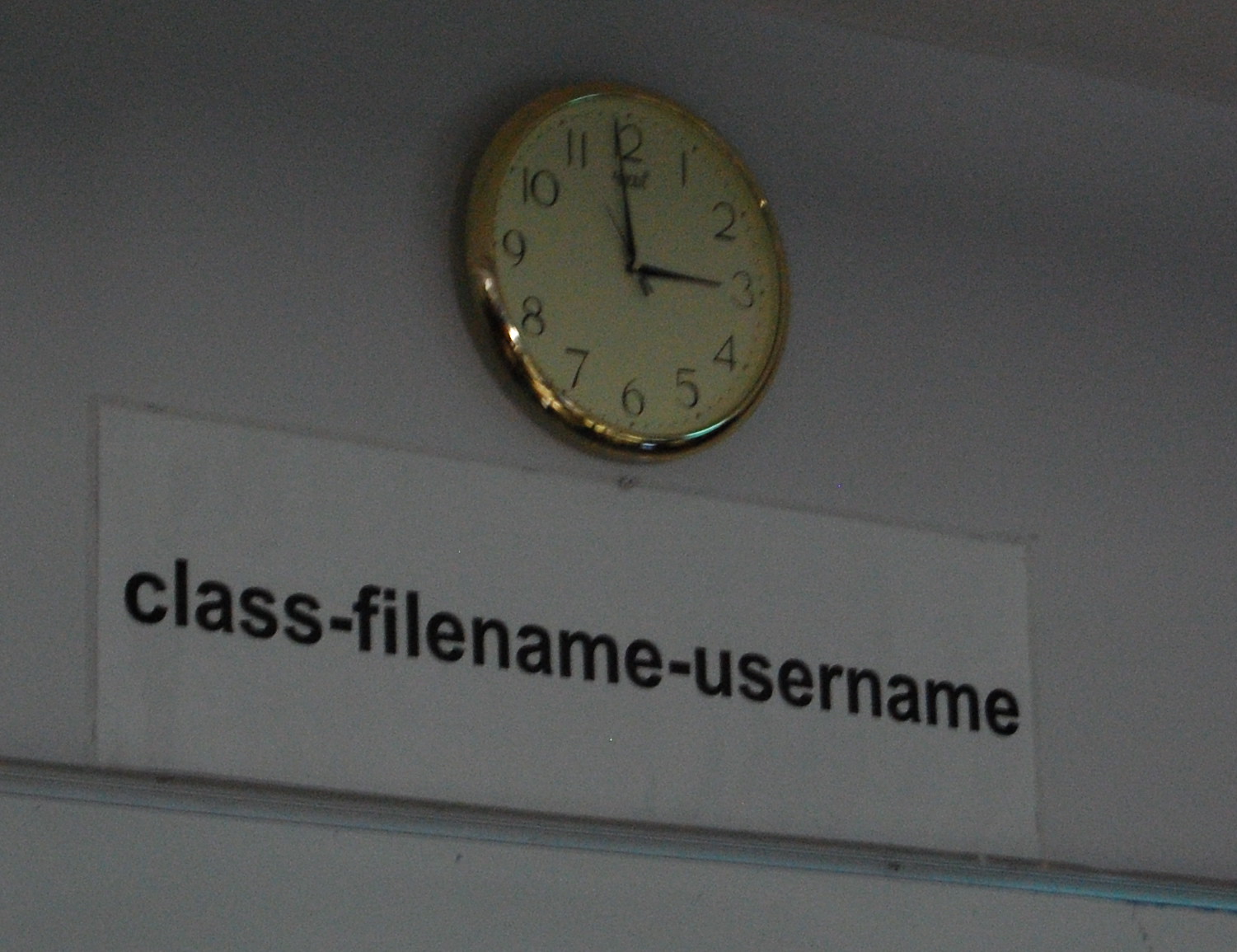This image depicts a section of a classroom interior, focusing on an area near the top of the wall close to the ceiling. A prominent clock, featuring a tan face and hands encased in a gold brass trim, is mounted above a doorway. The time displayed on the clock is 2:59. Directly beneath the clock, a white sign bears the text "class.-filename-username" in bold, black letters. This sign is positioned on a ledge, adding a sense of organized structure to the room's decor. The overall setting suggests a well-maintained academic environment.